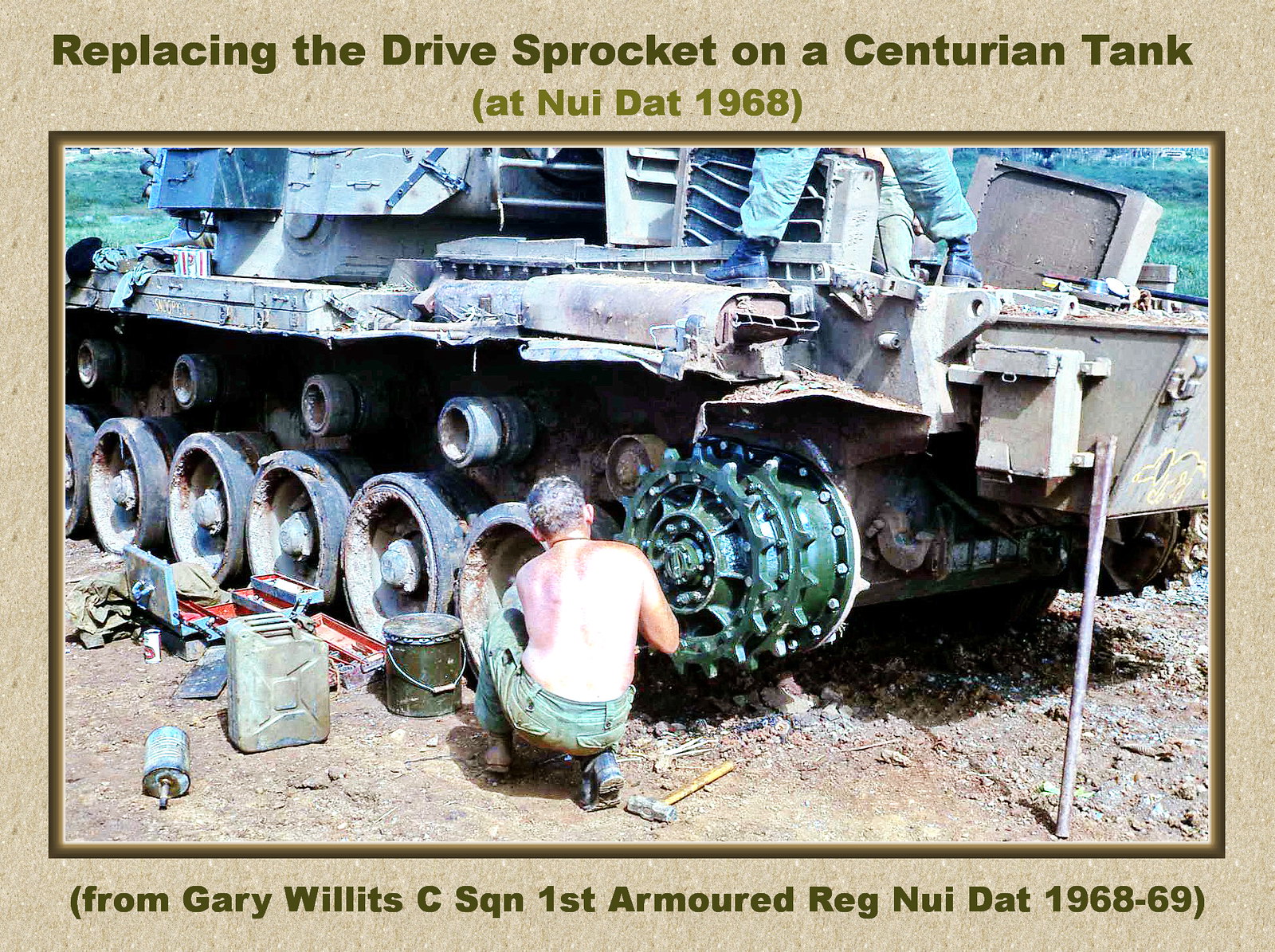This color photograph, framed with a beige border, captures a scene from 1968 at Nui Dat during the Vietnam War. The image shows a shirtless man in army green cargo pants and black boots, crouched down and working on the drive sprocket of a Centurion tank. He is facing away from the camera, intensely focused on his task. Surrounding him on the dirt ground are various tools, including a green bucket, a jerry can, an open toolbox, and a large sledgehammer positioned behind his back. The tank, which has six wheels on each side and a main wheel visible at the front, has its treads removed, exposing the inner parts. Additionally, a second serviceman, whose legs are straddled over the front edge of the tank, is partially visible as he stands on top of the vehicle. The scene is illuminated by daylight. The top of the photo reads, "Replacing the drive sprocket on a Centurion tank at Nui Dat, 1968," while the bottom notes, "From Gary Willett, C-Squadron, First Armored Regiment, Nui Dat, 1968-69."